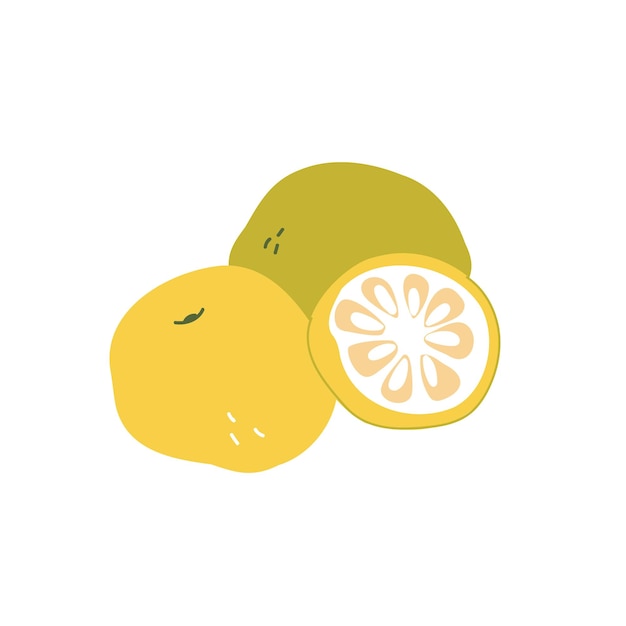This illustration depicts three imperfectly shaped lemons against a minimalist white background. The fruits, drawn in a simple, almost childlike style, vary slightly in color and form. On the bottom left, there's a dull yellow lemon with a small black mark near its base. Directly to its right is a lemon cut in half, revealing a white interior with eight seeds and a yellow outline. Behind these two lemons is another one with a greenish-yellow hue, adorned with three small marks. The drawing's simplicity highlights the lumpy, asymmetrical forms of the fruits, giving it a unique, rustic charm.